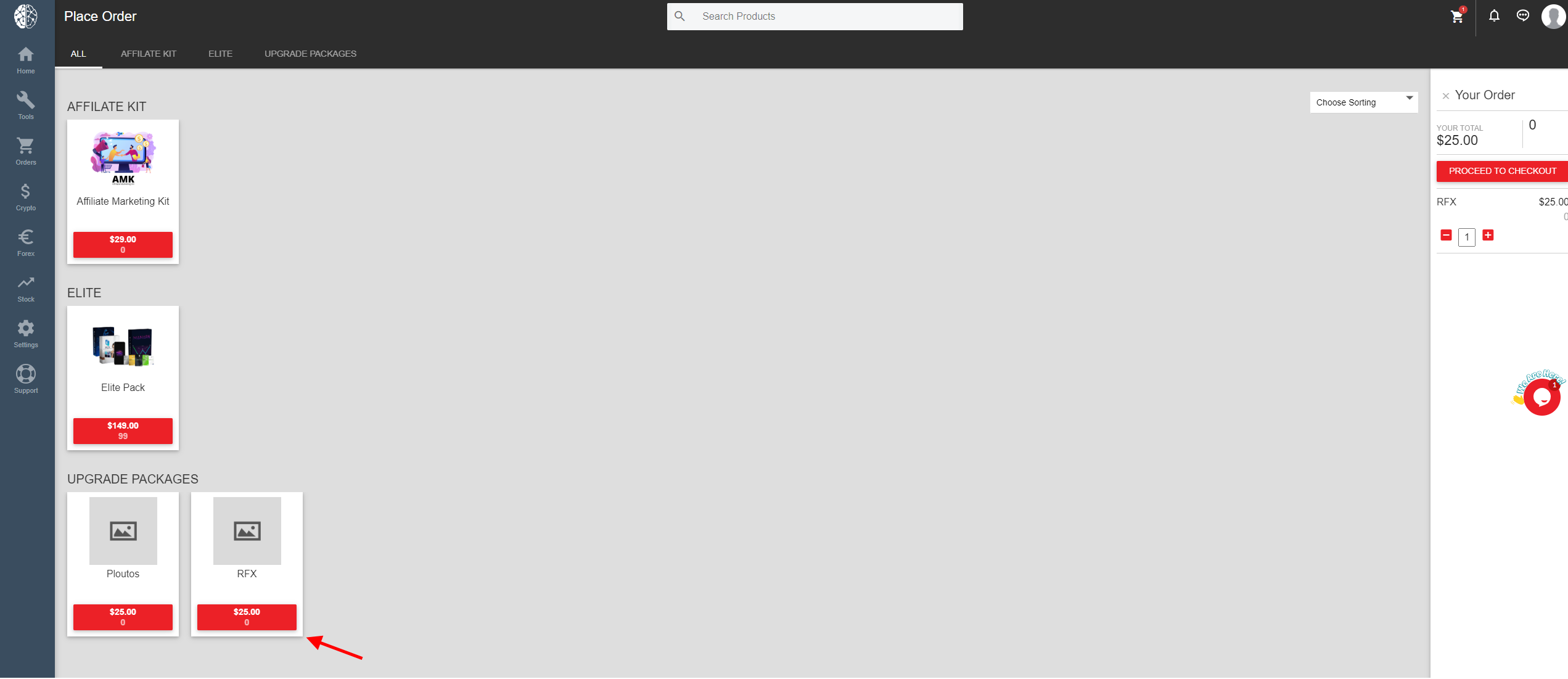Here's a cleaned-up and detailed caption for the image based on the provided description:

---

Screenshot of a digital interface with a black navigation bar across the top. The text "Place Order" is visible in the navigation bar. Below it, there is a prominent white section with a search icon, indicating a search functionality. On the left-hand side, there is a vertical menu with various gray icons. These icons include common ones such as "Settings," "Home," and a "Dollar Sign," among others that are not easily recognizable. One of the icons may indicate battery status. Within the main content area of the screenshot, there is a gray box featuring text that reads "Affiliate Kit" and "Elite Upgrade Packages."